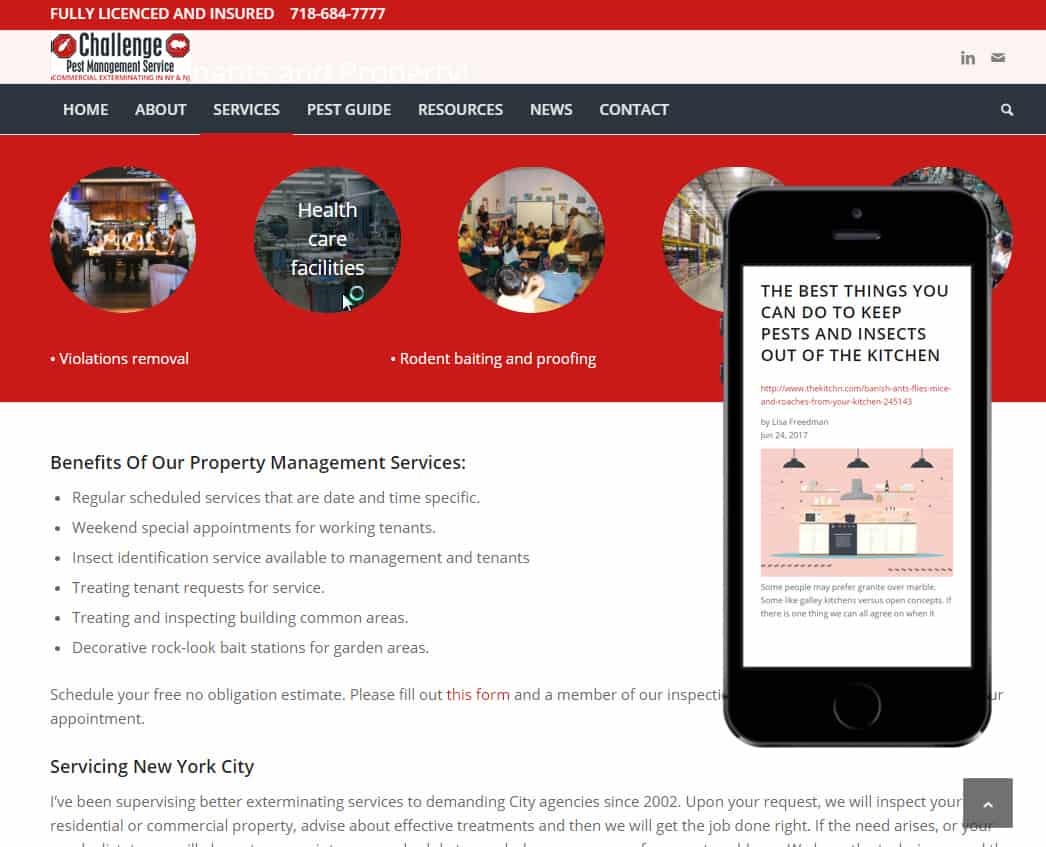This detailed caption describes a densely packed and commercial web page dedicated to pest control services.

---

The image is a screenshot of a predominantly commercial web page. The topmost section features a striking red bar with bold, white text declaring "Fully Licensed and Insured" alongside the contact number "718-684-7777." Directly below this, a white bar showcases the word "Challenge" in blue, followed by a very dark gray bar. This gray bar contains navigational options in white font, including "Home," "About," "Services," "Pest Guide," "Resources," "News," and "Contact," with a small white magnifying glass icon signifying a search function at the far right end.

Further down, a vivid red bar displays five circular thumbnails containing images too small to discern. Below these images, the text in white reads "Violations Removal, Rodent Baiting and Proofing." Overlaying the final two circular images is a graphic representation of a smartphone with black bezels. The phone's white screen displays text stating, "The best things you can do to keep pests and insects out of the kitchen," suggesting an article is open below, with content too small to read.